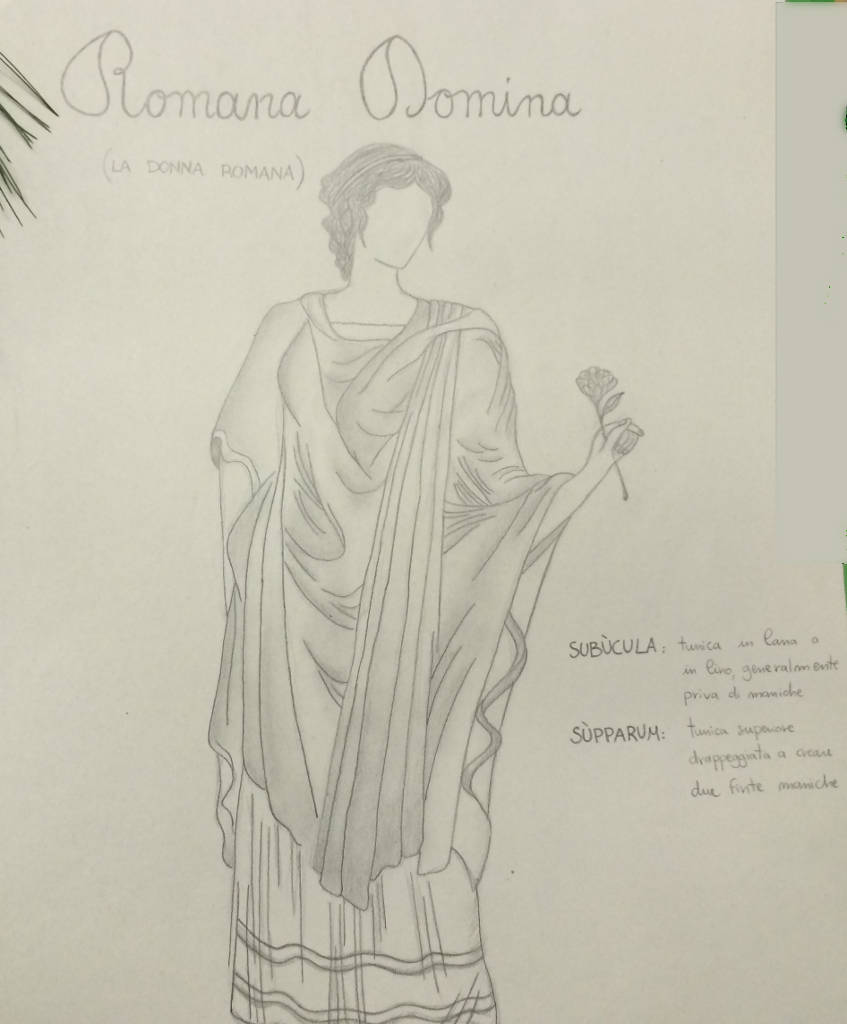This sketch, titled 'Romana Dominia' with the parenthetical note 'Ladonna Romana', depicts a woman adorned in traditional Roman attire. She is portrayed with one hand elegantly tucked into her flowing robes, while the other hand delicately holds a flower. The woman features short hair but notably lacks facial details. In the lower right corner of the sketch, the word 'Symbiocula' is inscribed, accompanied by some cursive text that remains indecipherable. Beneath this, 'Supartum' is also written, followed by additional cursive writing that is illegible.